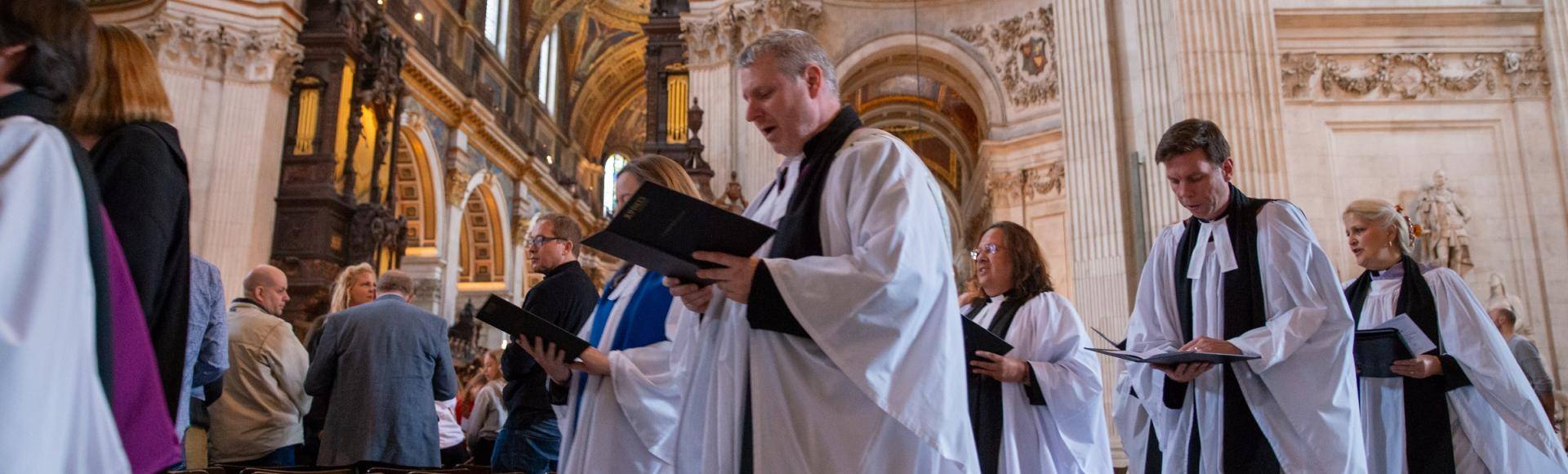The image depicts a long, narrow, panoramic view of a grand cathedral's interior during a church service. In the foreground, a procession of choir members is moving two by two, though it is unclear whether they are walking into or away from the choir loft. The choir consists of both men and women, all dressed in flowing white robes accented with black scarves around their necks. Some choir members also have two white strips of fabric tied around their necks, similar to a tie, and one woman notably wears a dark navy blue scarf. Each choir member holds a thin, black hymnal book, its pages open as they sing the hymns. Their facial expressions suggest they are deeply engaged in the performance. Behind the choir, a minister and two other individuals in suits can be seen. The church’s interior is grand and ornate, featuring light tan stone walls, dark wood elements, and gold-painted decorations, evoking the traditional aesthetics of a Catholic Church. The background further reveals a congregation either entering or exiting, adding a dynamic layer to the solemn setting.